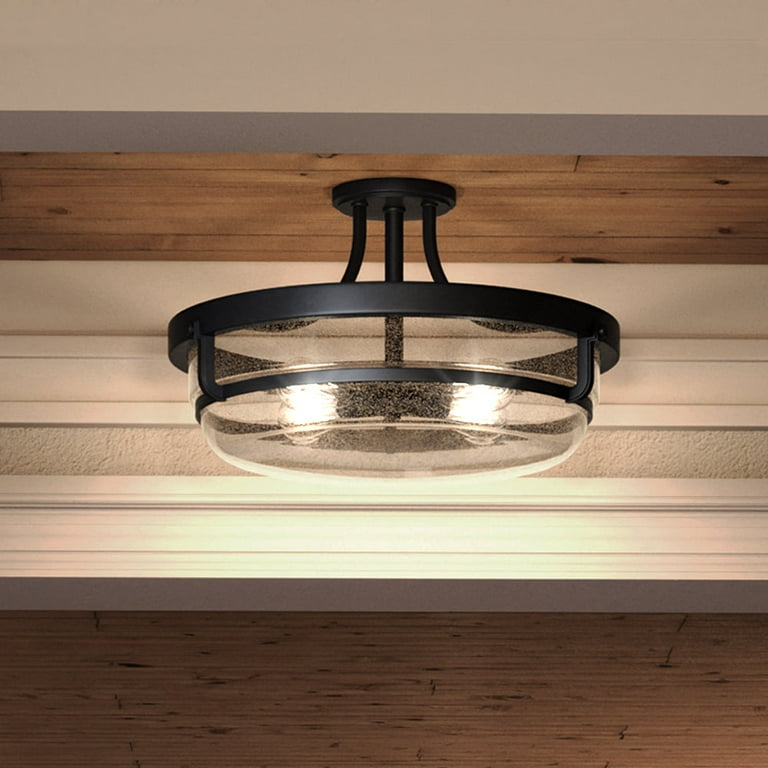The image captures a close-up, square-shaped photograph focusing on a semi-flush mount light fixture attached to a ceiling with a wood effect. The ceiling consists of medium brown wooden planks. Towards the foreground, there's a creamy green soffit separating the wooden panels from additional ceiling elements. The light fixture itself features a black ceiling rose and a black pole leading down to a speckled clear, seeded glass fitting. This glass enclosure, showing two visible bulbs, is encased in a distinct metal frame with both thicker and thinner elements connected by vertical pieces spaced evenly around its circumference. The background showcases a mix of creamy green, white, and tan molding, adding to the aesthetic contrast and highlighting the fixture. The composition gives an impression of a professional product photograph, possibly designed for a home goods catalog.